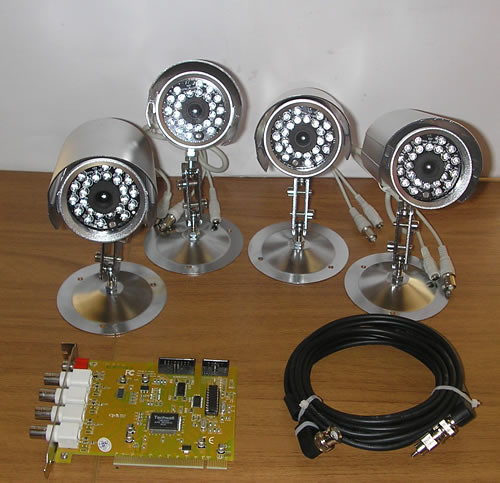This color photograph captures a set of four spotlight-like objects prominently arranged on a dark brown wooden surface, with the wood grain running horizontally. Each light features a wide, circular base transitioning into a slender, silver metal stem. Atop each stem is a conic-shaped fixture housing small, white lights, reminiscent of spotlights or Pixar-esque lamps. Behind the objects, the upper third of the image is filled with a grey background that displays subtle shading on the right side.

A rolled-up black power cord, secured with small white plastic ties, is placed in the bottom right corner. This cord has metallic connectors on both ends, with the left connector being flat and silver, while the right one appears rounded and white. To the left of the black cord lies a green circuit board, notable for its several small metal rectangular protrusions and four white ports with metallic elements. A small red component is visible in the top left corner of the circuit board. The photograph is well-lit, emphasizing the sharp details and varied textures of each element.